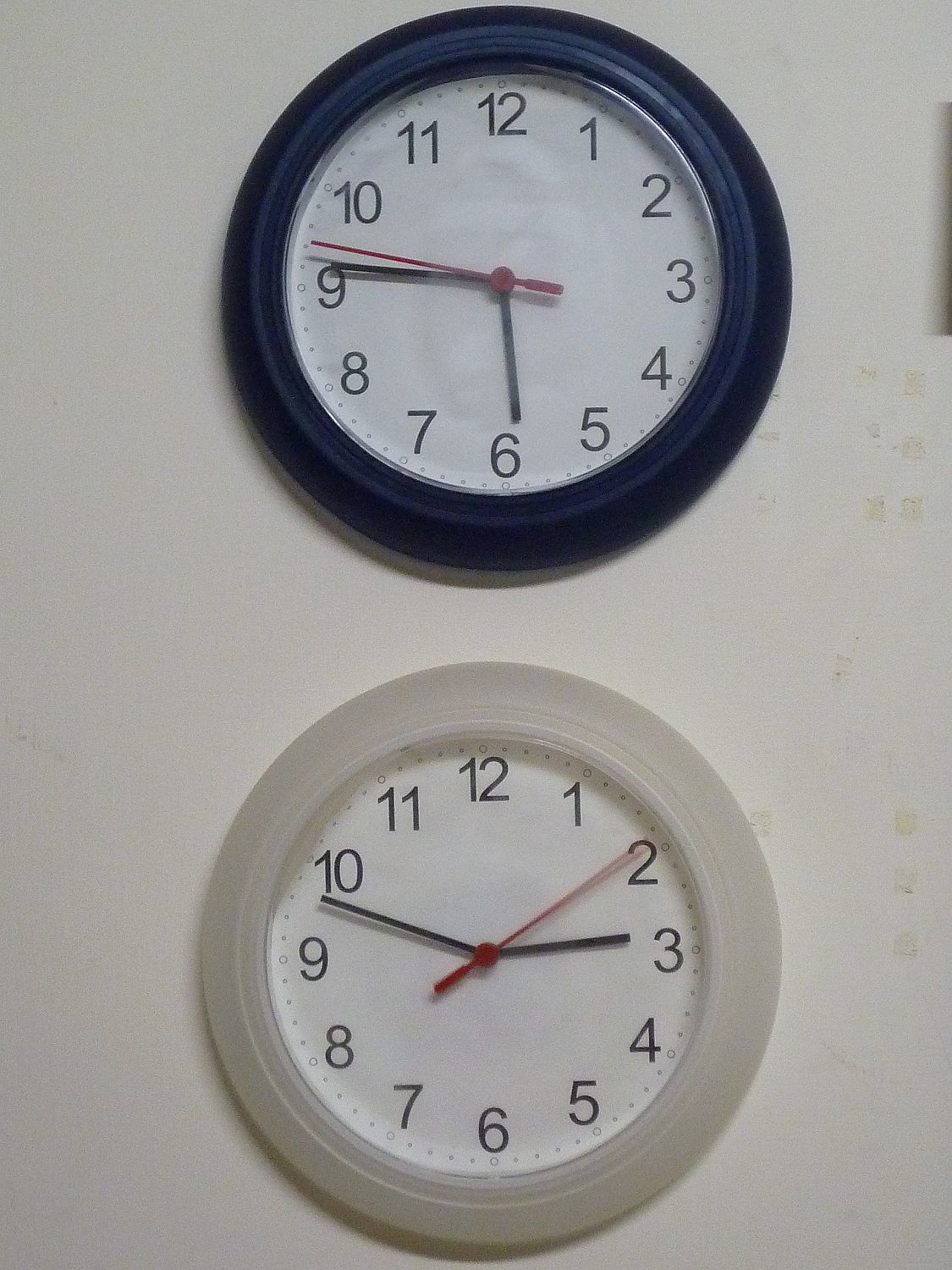The image features two clocks mounted vertically on a white wall. The wall shows some minor markings, possibly from tape residue. Both clocks appear to be from the same manufacturer, with a diameter of approximately 10 to 12 inches each. The top clock has a dark blue, beveled frame, while the bottom clock has an off-white, beveled frame. Each clock has a white face, black sans serif numbers, and three hands: an hour hand, a minute hand, and a red second hand. For the top clock, the time reads about 5:46, with the second hand at 48 seconds. The bottom clock displays the time as approximately 2:48, with the second hand at 9 seconds.